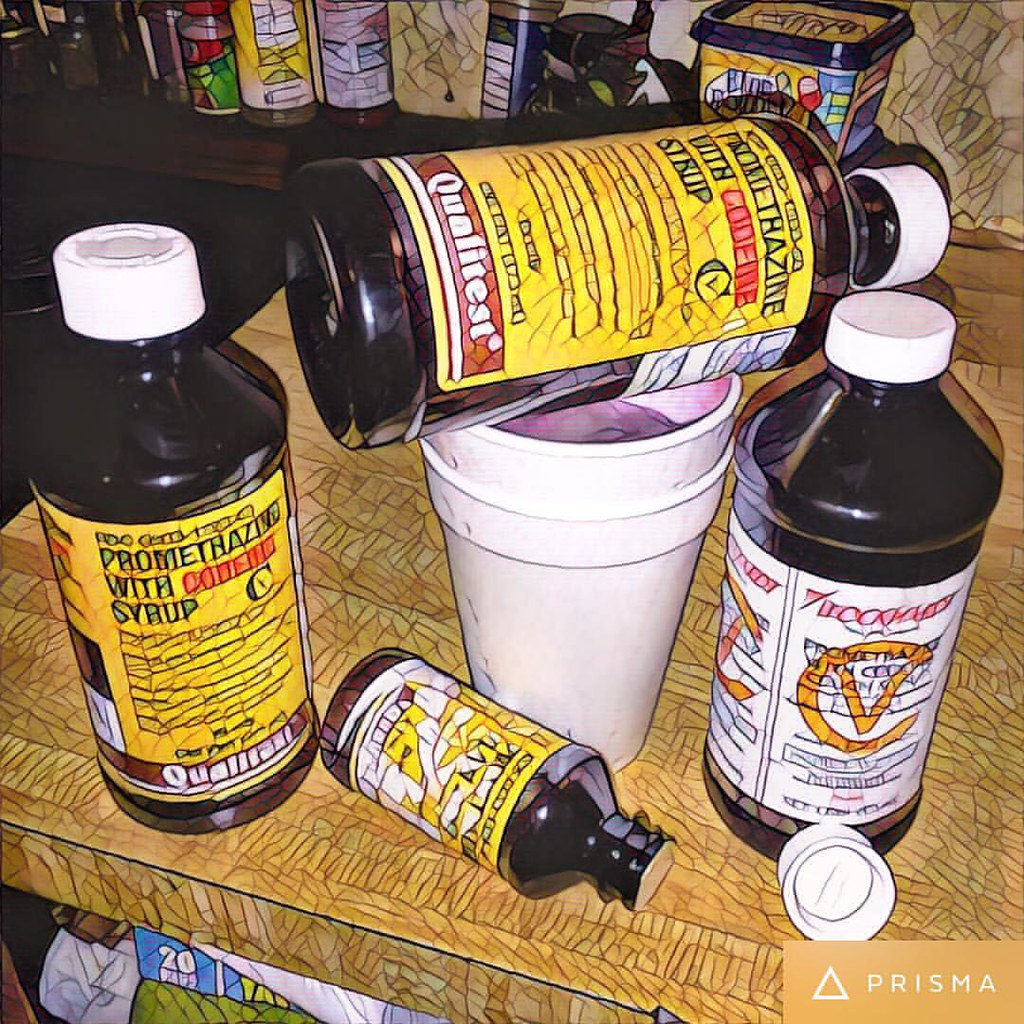This image has been artistically manipulated using a Prisma filter, imparting a hand-drawn, colored pencil effect while retaining its photographic origins. At the bottom right corner of the image, the Prisma logo confirms the filter application. The main focus is four prominent bottles – likely containing promethazine cough syrup – placed on an aged, chipped Formica countertop. Two of the bottles stand on either side of a pair of stacked white styrofoam cups, the uppermost cup showing a purple liquid inside, suggestive of its content. One bottle lies on its side in front of the cups, with its childproof cap unscrewed and resting against another bottle. Below the counter, a partially visible plastic wrap roll can be seen, along with an array of different household products arranged on a shelf. The setting appears to be a cluttered kitchen, underscored by a dark brown background with bottles of spices and other cooking containers lining a ledge. The overall combination of cough syrup bottles and the telltale purple liquid evokes connotations of recreational use.